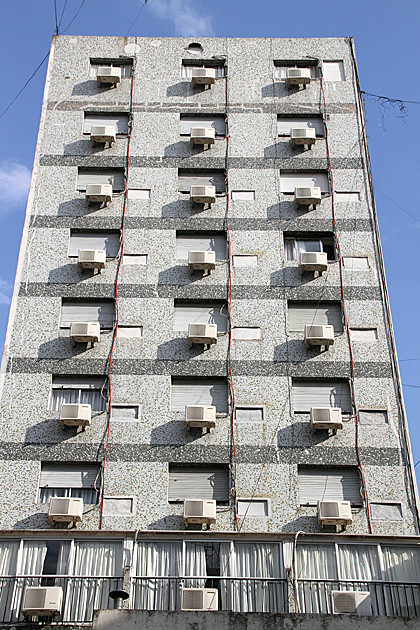The photograph features a tall apartment complex or hotel spanning approximately eight or nine stories, predominantly occupying the frame. The building is constructed from speckled light gray concrete with darker gray horizontal stripes accenting each row of windows. There are 21 small, square windows with white horizontal blinds, each fitted with an external box air conditioner. The ground floor deviates with wider sliding glass doors, adorned with curtains, and includes a small balcony, separated from the upper floors by their distinct window style. Large electrical cables, in columns, run vertically along the sides of the structure, presumably providing power to the air conditioners. Framing a bright blue sky with wispy white clouds, the background adds to the sense of a sunny day. In the foreground, a fence or balcony is visible, marking the boundary from the viewer's vantage point.